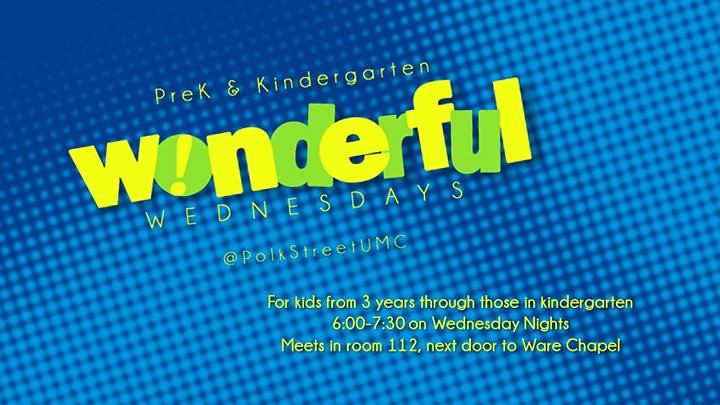This is a rectangular-shaped poster with a dynamic blue background featuring a checkered pattern in dark and light blue shades. Prominently displayed at the top of the poster is the word "WONDERFUL" in large letters, with each letter alternating between yellow and green colors. Above this, in smaller yellow text, reads "PREK AND KINDERGARTEN." Below "WONDERFUL," the text "WEDNESDAYS" is positioned. An additional detail includes the letter 'O' in "WONDERFUL," which creatively contains an exclamation mark. Towards the lower part of the image, the text in yellow reads, "For kids from 3 years through those in kindergarten, 6:00 - 7:30 on Wednesday nights. Meets in Room 112 next door to Ware Chapel." This appears to be an advertisement for an event at Polk Street UMC, specifically designed for young children.